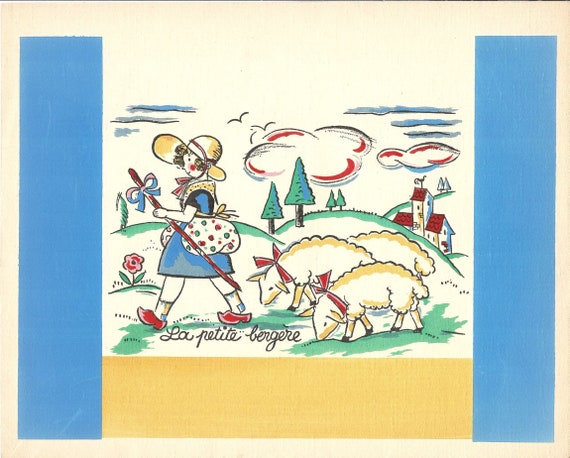In the center of this color illustration, a young girl, seemingly a shepherdess, is depicted leading a small flock of sheep. She is dressed in a striking blue dress paired with a white apron adorned with charming black and green dots. Her broad-brimmed yellow straw hat shields her from the sun, while her feet are shod in distinctive red wooden clogs. The shepherdess also carries a brown stick, elegantly adorned with a blue ribbon tied in a bow at the top. Her sheep follow obediently, each with a red ribbon tied in a bow around their necks.

The background of the image reveals a scenic countryside with gentle rolling hills, trees, and a charming building featuring a red roof and a rooster perched atop it. Overhead, clouds outlined in red and blue float through the sky, accompanied by a few birds. The entire scene is framed by vertical blue bands on both sides and a horizontal yellow band at the bottom. Below the illustration, in graceful black cursive, the text reads "La Petite Bergère," adding a touch of elegance to this whimsical portrayal. The off-white background provides a gentle contrast to the vibrant colors of the illustration, suggesting it may be part of a children's book.